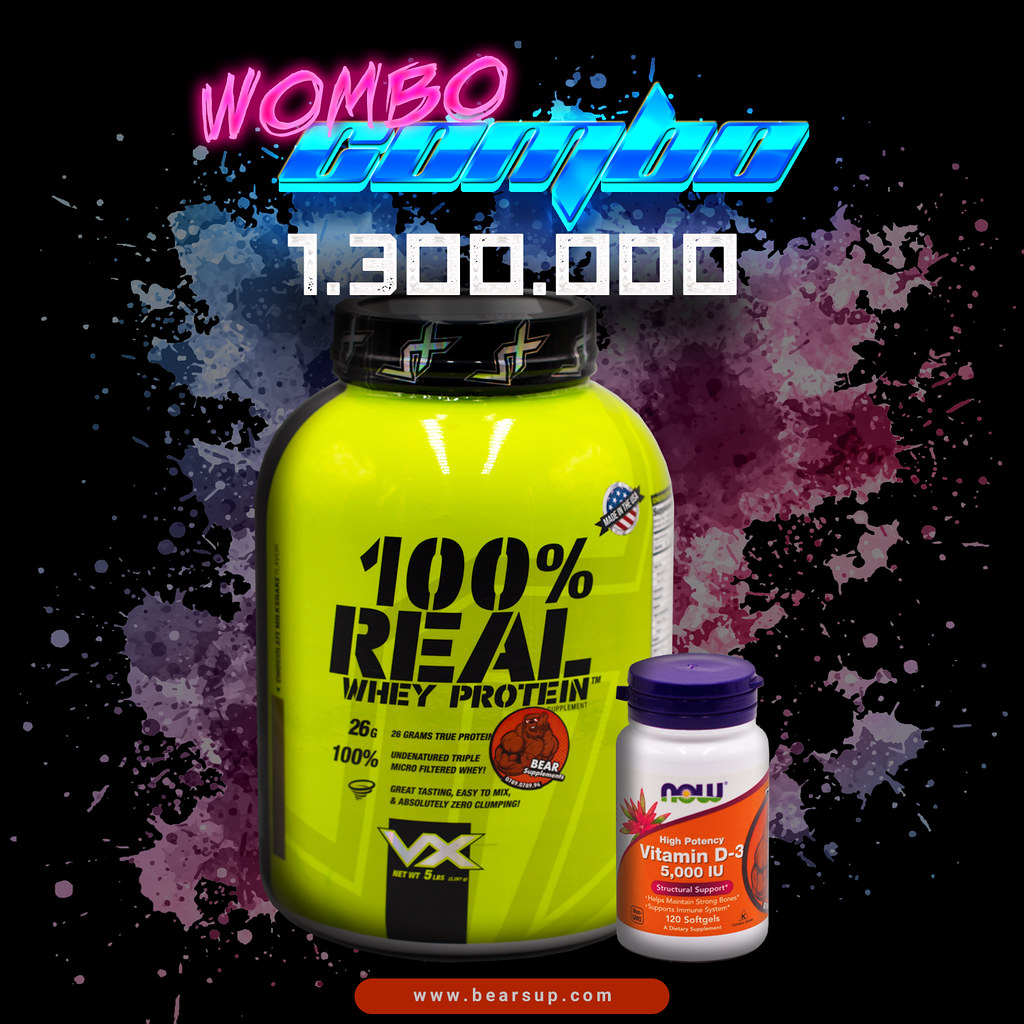The image is a detailed advertisement poster likely seen in a retail store, featuring a striking black background with an abstract, nebula-like design at the top. Prominently displayed at the top in bright colors are the words "WOMBO" in hot pink and "COMBO" in blue. Below this, a large white number "1.300.000" stands out. Centered in the image is a large yellow container prominently labeled "100% real whey protein" in bold black print. Detailed descriptions tout it as containing "26 grams true protein," being "100% undenatured triple microfiltered whey," and emphasizing its "great tasting, easy to mix, and absolutely zero clumping" qualities. Next to the protein container is a smaller bottle of vitamin D3 from Now Foods, characterized by a blue top, white upper half, and orange lower half, clearly labeled "5000 IU." At the bottom of the poster is the web address "www.bearsup.com" and a logo in a black oblong shape with "VX" in white letters, representing the brand. The entire layout is set against a colorful, almost spilled-paint-like splotch of colors, further enhancing its vibrant and eye-catching appeal.